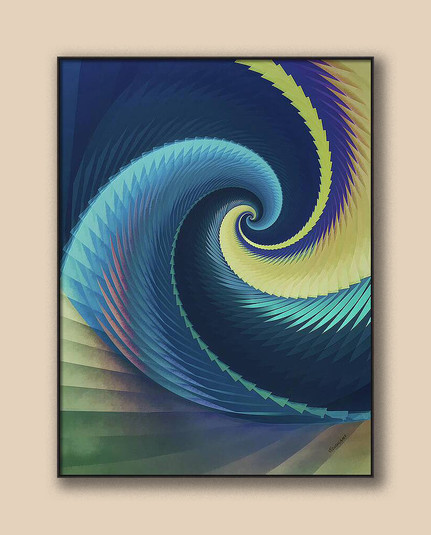The image is a vertically oriented, rectangular painting set against a tan-colored wall. It features a thin black frame that accentuates its modern design. The artwork itself depicts a dynamic and visually captivating scene composed of large, swirling wave shapes that intertwine gracefully. Dominant colors in the painting include diverse shades of blue ranging from dark to light, alongside vibrant golds and subtle hints of green, pink, violet, and maroon. 

At the bottom of the painting, there is a section resembling a staircase or stepped platform, starting flat and ascending in a brown hue with touches of green. Above this, a prominent wave shape unfurls, curling elegantly in the center with a palette of blues, greens, and a splash of pink. Another wave, primarily gold and violet, descends from the upper right, intersecting with the central wave. In the upper left corner, a darker blue wave adds depth and balance, also curling towards the middle like the others.

Additionally, amidst the swirling colors, there's emphasis on the spiral formations and thin lines in various hues, including a thinner maroon line next to a light blue section toward the bottom. Small arrow-like shapes in green are interspersed within these spirals, adding further intricacy to the overall composition.